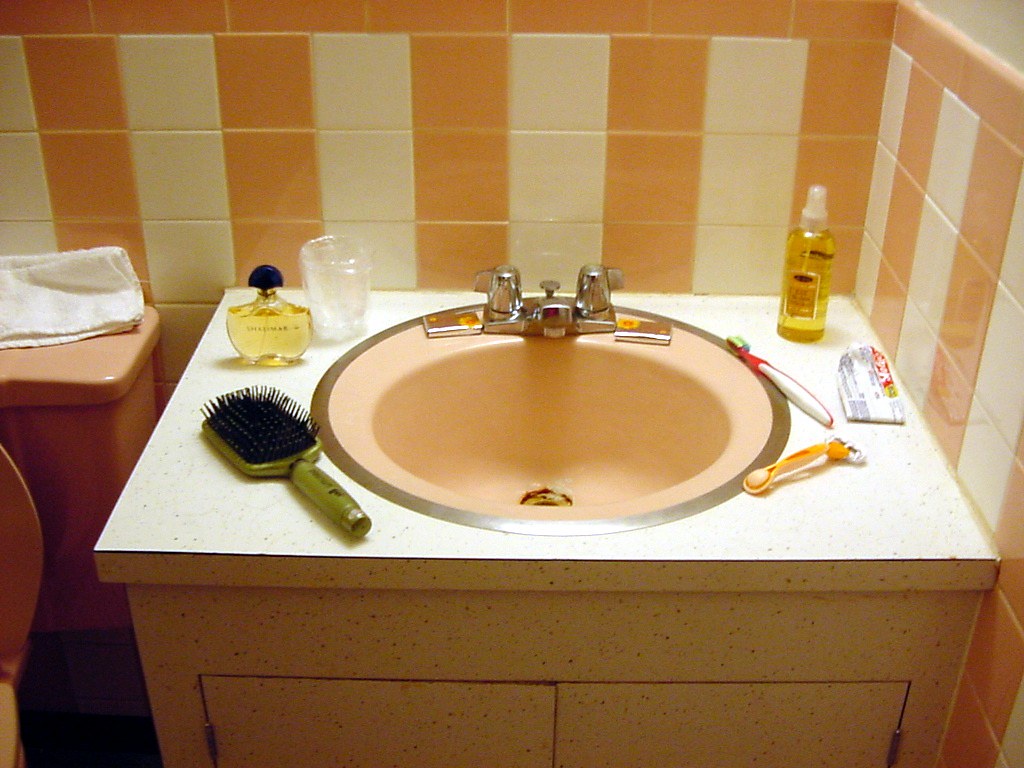A detailed close-up image of a standalone vanity in a bathroom showcases a unique, melon-colored finish on the cabinet that resembles sandstone with a grainy texture. This finish is accentuated by an array of dark brown and light tan specks, as if the surface was artfully splattered with multiple colors. Behind the vanity, an orange and cream-colored striped wall features wide, vertically-arranged tiled stripes that extend from the ceiling to the floor. These cream stripes harmonize with the creamy tan-colored, silver-outlined sink that showcases a sleek white Formica top. In the bottom left corner of the image, a toilet and its tank are visible, both coordinating with the vanity and the cream hues in the striped wall. On the vanity countertop, specific items are placed in a thoughtful arrangement: a brush at the 8 o'clock position, a couple of bottles of cologne at the 10 o'clock position, and a razor at the 4 o'clock position, adding a personal touch to the pristine bathroom setting.